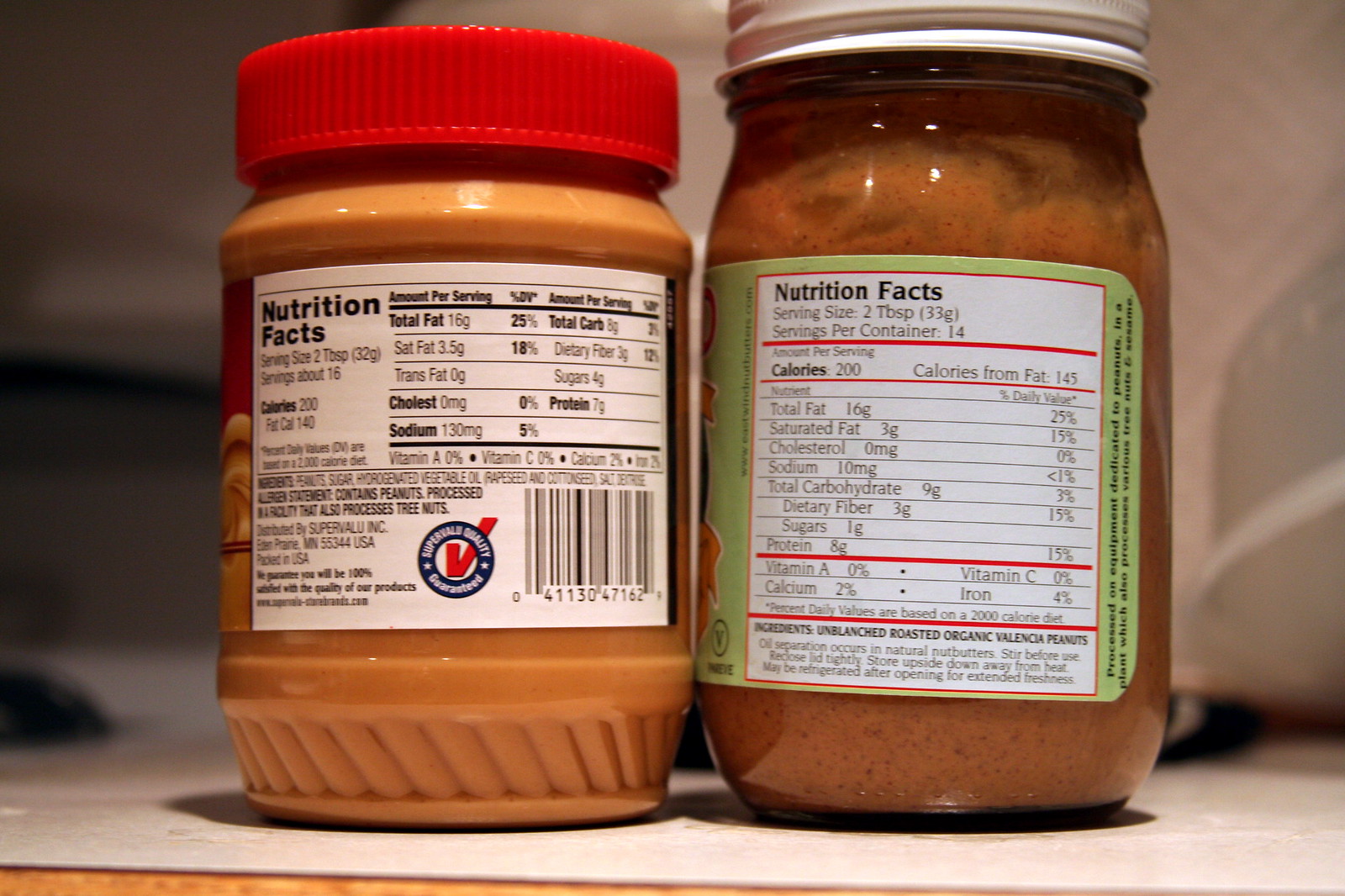This horizontal close-up photograph features two jars of peanut butter, focusing on their nutritional facts. The jar on the left contains a two-tablespoon serving with the following nutritional values: 200 calories, 140 of which are from fat, 16 grams of total fat, 3.5 grams of saturated fat, zero trans fat, zero cholesterol, 130 milligrams of sodium, zero carbohydrates, 3 grams of dietary fiber, 4 grams of sugar, and 7 grams of protein. Its ingredients include peanuts, sugar, hydrogenated vegetable oils (rapeseed and cottonseed oil), and it is processed in a facility that handles tree nuts. The jar is distributed by Super Value and also features a barcode.

The jar on the right provides nutritional information for a two-tablespoon serving with 200 calories, 145 of which come from fat. It contains 16 grams of total fat, 3 grams of saturated fat, zero cholesterol, 10 milligrams of sodium, 9 grams of total carbohydrates, 3 grams of dietary fiber, 1 gram of sugar, and 8 grams of protein. Additionally, this peanut butter offers 0% of the daily value for vitamin A and vitamin C, 2% for calcium, and 4% for iron. The ingredients include unsalted, roasted, organic Valencia peanuts and the label advises consumers to stir before use, indicating that it is natural peanut butter. Some parts of the label appear blurry.